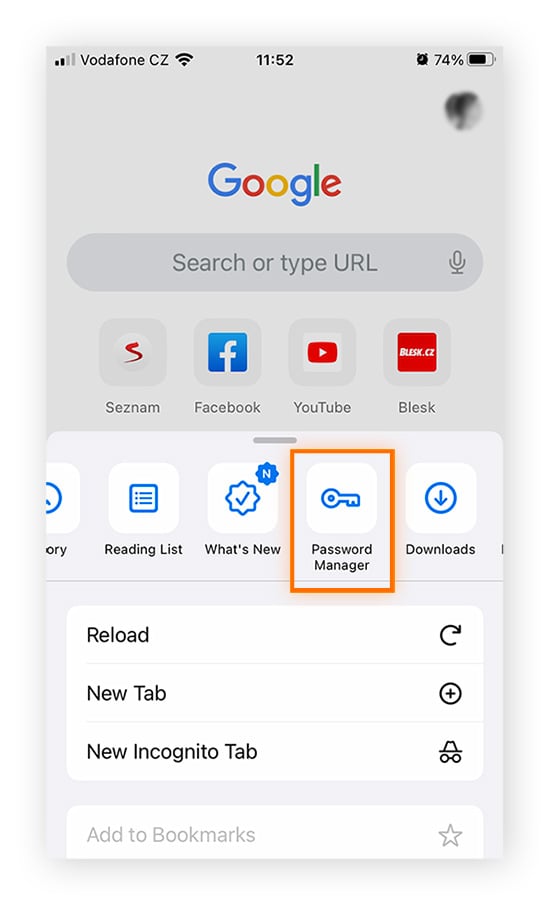This image is a cropped mobile screenshot showcasing the Google homepage. Centered at the top of the screenshot is the colorful Google logo, followed directly underneath by the familiar search bar. The search bar contains the grey placeholder text, "Search or type URL." Positioned below the search bar are four icons representing frequently visited sites or saved bookmarks: the first reads "SESNAM," followed by icons for Facebook, YouTube, and Blesk.

Towards the bottom of the screenshot, a pop-up box appears overlaying the screen, displaying a list of icons in blue. These icons are labeled "Reading list," "What's new," "Password manager," and "Downloads." Notably, the "Password manager" option is enclosed within a red box, seemingly edited into the photo to highlight it as a focal point for instructional purposes. At the very bottom of this pop-up, options for "Reload" and "New Incognito Tab" are visible. Additionally, "Add to bookmarks" is present but greyed out, indicating it is currently unavailable.

In the top left corner of the screenshot, it is evident that the person who took the screenshot is signed into their Google account, though their profile photo has been pixelated to obscure their identity.